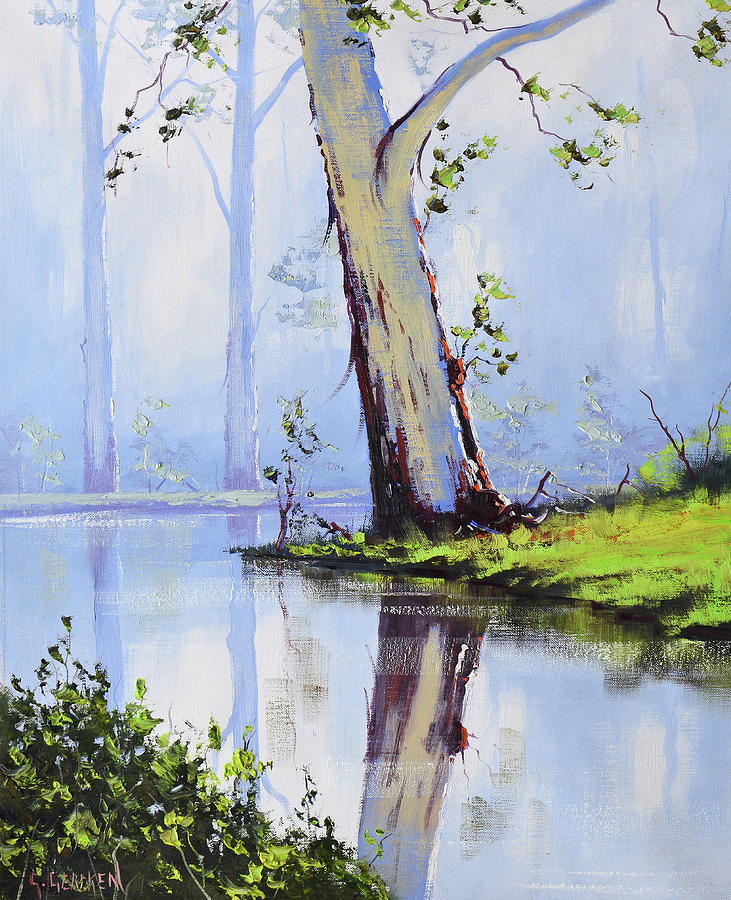This is a detailed painted illustration in portrait mode, featuring a serene, ethereal landscape dominated by a gently flowing river that winds its way through the scene. The river starts in the lower right corner, diagonally crossing towards the left, then bending right again into the distance, forming a soft 'C' shape. The water is a light, pastel blue and reflective, mirroring the surrounding elements. At the very center stands a prominent tree, with a trunk and a few branches shooting upwards and outwards, towering too tall to capture its leafy canopy. This tree, with its blue, yellow, and hints of red bark, creates a focal point, leaning slightly, with the impression of someone sitting against it, though it's not entirely clear.

In the far end of the river, there are two white and light blue trunks, likely birch trees, similarly reflected in the water. Bright green grass carpets the ground, spreading from the right bank of the river to the lower left corner where a lush bush adds to the verdant scenery. The overall palette of the painting includes pastel colors, with bright greens and a pervasive blue tint, giving the whole image an unreal, almost surreal quality.

The artist's signature, "L. Bleethan," marked in pink or reddish stylized lettering, is located in the bottom left corner of the painting. The harmony of colors and reflections enhances the painting's tranquil beauty.